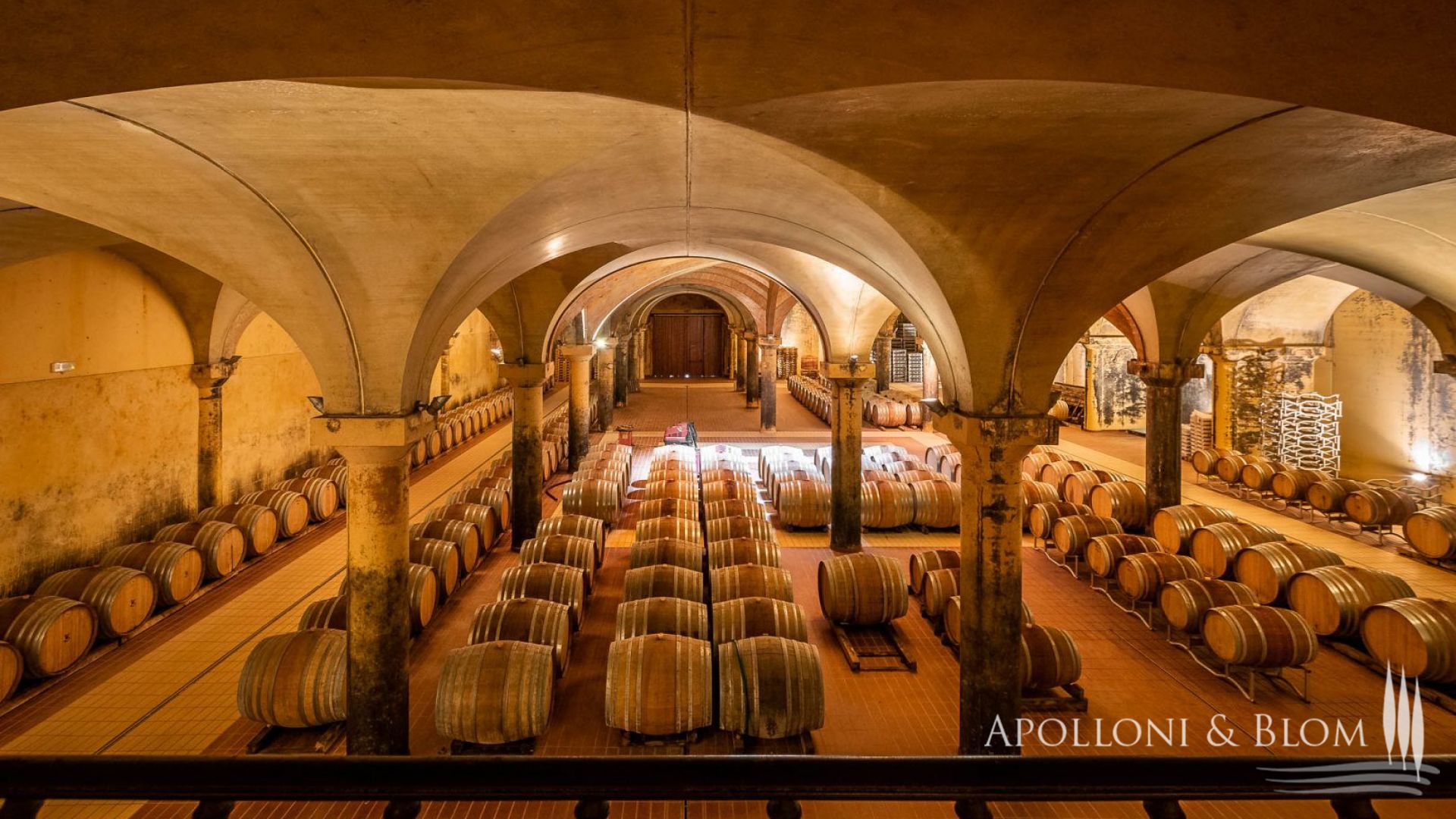This photograph captures the interior of an expansive and meticulously organized wine cellar or storage room, likely part of a vineyard or winery. The room features a high vaulted ceiling made of a smooth beige material, supported by pillars that are worn at the base, transitioning from beige at the top to dark gray or black towards the bottom. The ceiling arches elegantly between these cylindrical pillars, enhancing the grandeur of the space.

The cellar floor is clean and tiled with beige bricks, forming distinct pathways between rows of barrels. Parallel rows of medium brown oak barrels with gray metal bands are neatly arranged along the worn beige walls and spill into multiple rows extending towards the center of the room. A bright white light illuminates this central area, shining down onto the barrels, emphasizing their orderly placement and the cellar’s architectural details.

In the bottom right corner of the image, there is white text that reads "Apolloni and Blom," accompanied by a stylized logo featuring three cypress trees above three horizontal streaks representing the ground. The walls appear to be constructed from stone or cement, suggesting a historic or well-established facility. The overall scene is framed as though the photo is taken from an elevated perspective, adding to the depth and comprehensiveness of the room. The purpose of this cellar is clearly the aging and fermenting of wines or other alcoholic beverages, as suggested by the numerous oak barrels distributed throughout the space.